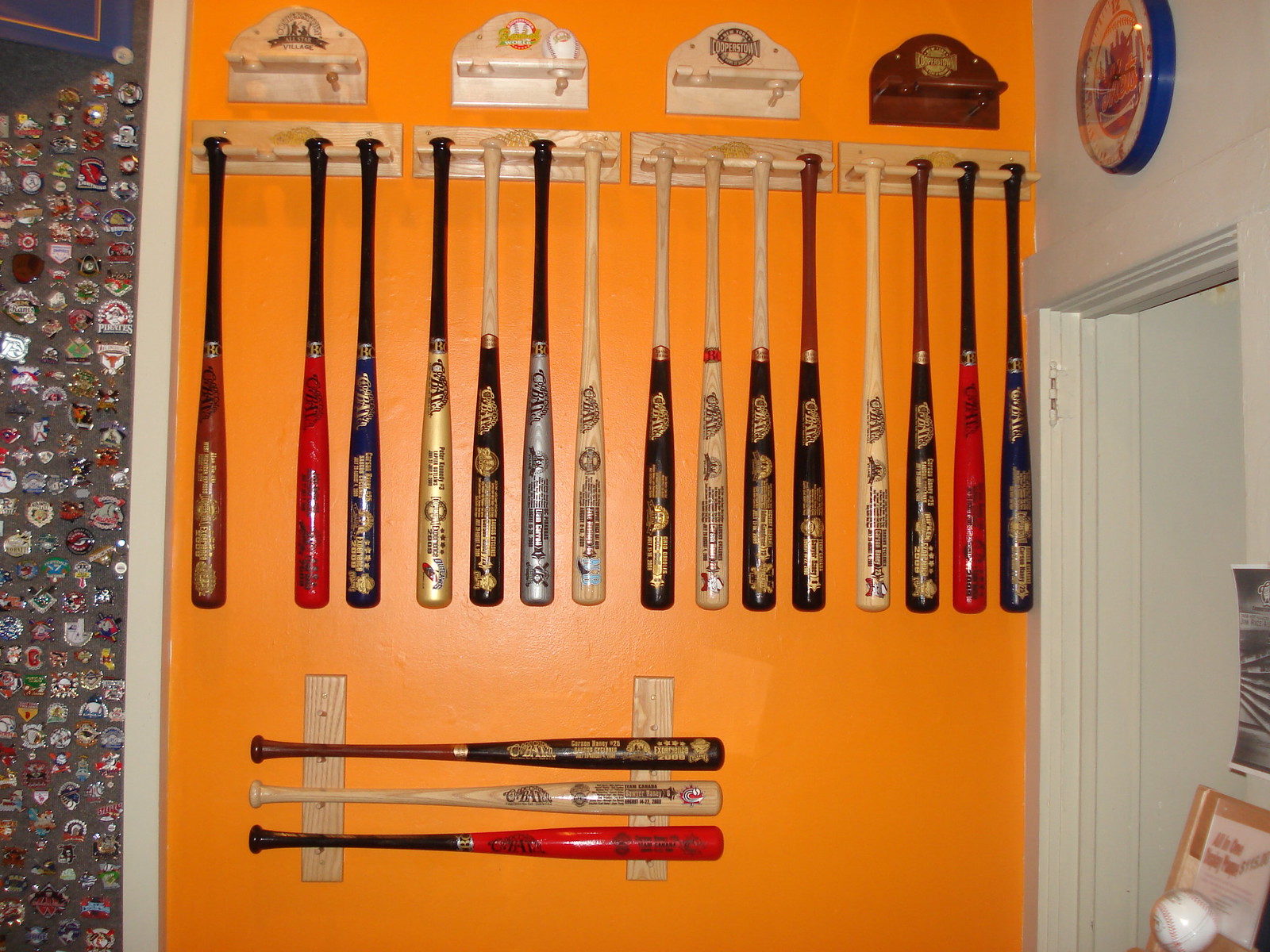This detailed image captures a well-organized tribute to baseball, prominently displayed on an orange-painted wall. The centerpiece features four wooden bat racks mounted high on the wall, each designed to hold four baseball bats upside down. Notably, one slot in the leftmost rack is empty, leaving a total of 15 bats displayed. The bats come in various colors, including black, red, tan, silver, and raw wood, and some feature extensive painted designs, possibly from different leagues. Below these, another set of bat holders made up of two vertical bars supports three bats laid horizontally.

Above the main bat racks, three additional empty bat holders and a small shelf-like space adorned with logos can be seen. To the left of this arrangement, a narrow gray panel is densely covered with a multitude of refrigerator magnet-like patches and pins, running the full height of the wall.

On the right side of the image, near the front corner, a baseball is displayed inside a plastic case on a plaque, with a poster visible above it. A doorway with a barely visible clock positioned above it completes the scene, creating a rich and detailed visual tribute to various baseball memorabilia.